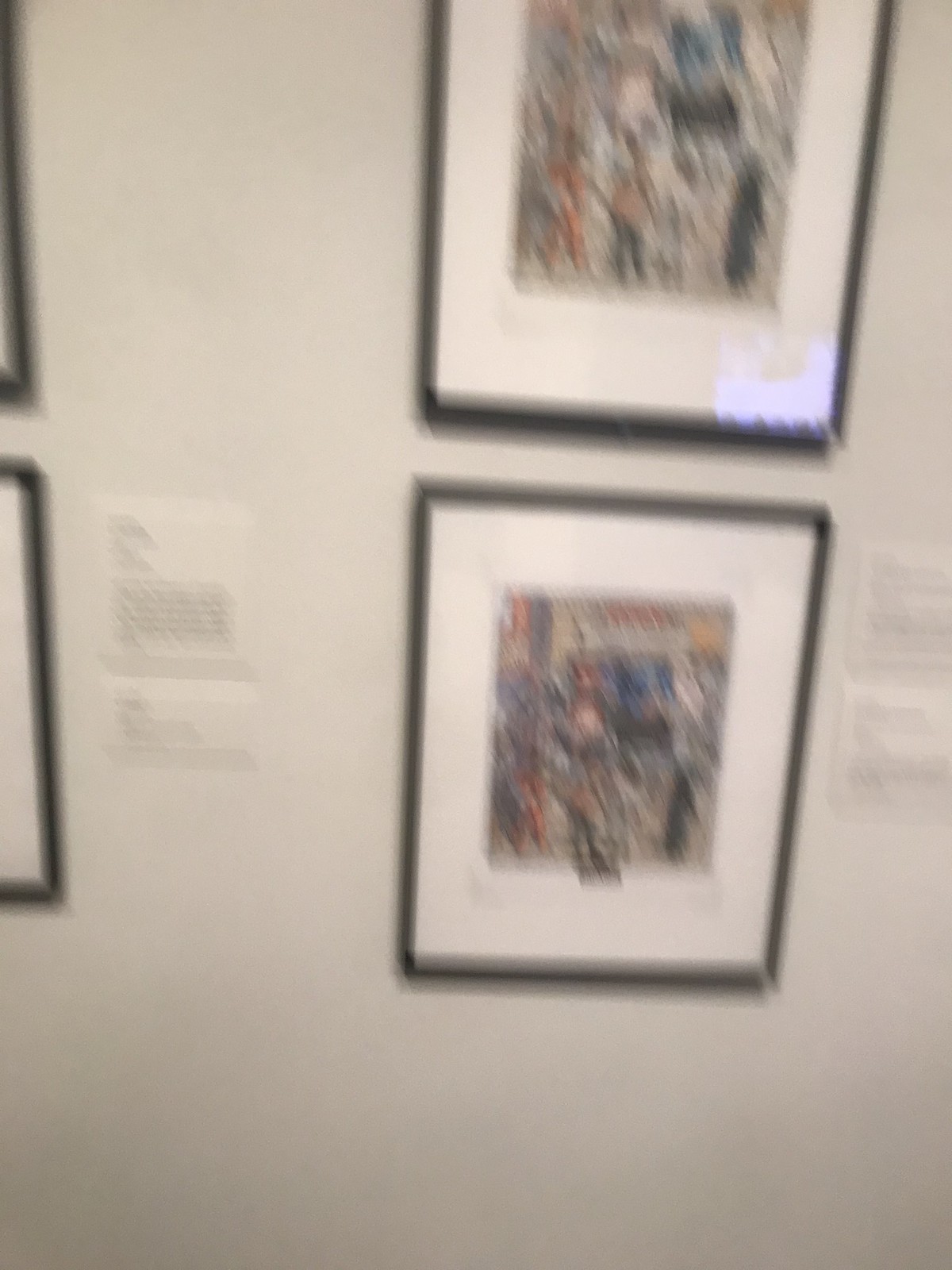This photograph captures a scene from an art gallery, depicting a section of a wall adorned with four black-framed artworks, possibly paintings or photographs. Each piece is centrally positioned within its frame and accentuated by a relatively thick white border. The image is notably blurry, likely due to camera movement during the shot, rendering the details of both the artworks and the descriptive plaques beside them indistinct and hard to decipher. Despite the lack of clarity, the general arrangement and presentation of the gallery wall are evident.